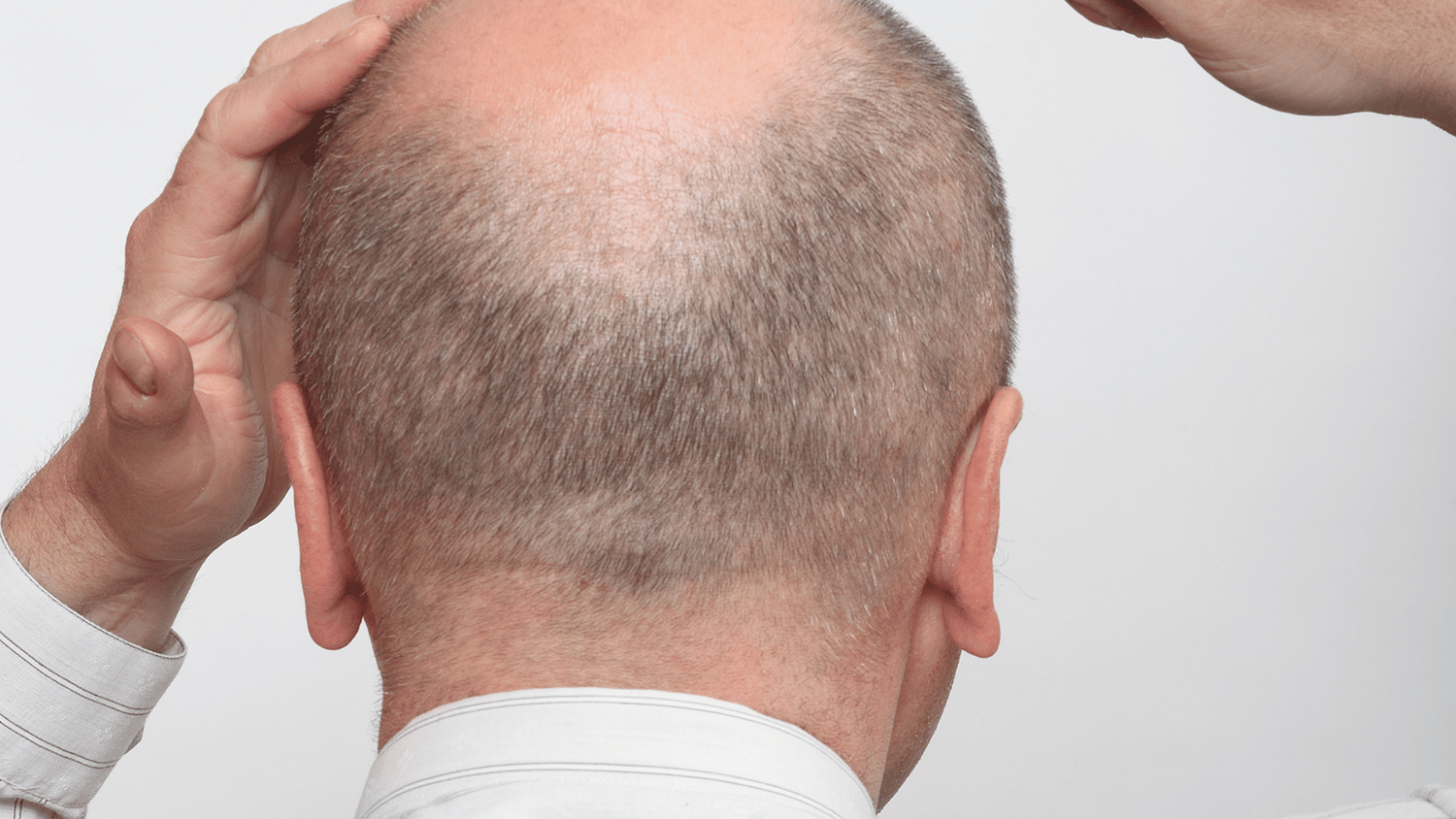This indoor color photograph is a close-up of the back of a balding white male, likely in his mid-40s. The image predominantly captures his head and upper neck, revealing light brown hair around the balding top. He wears a white collared dress shirt with small pinstripes and has well-groomed fingernails. His right hand is positioned just above his right ear, while his partially visible left hand appears in the top right corner of the frame. The man's ears, slightly pink and pointed backward, as well as a bit of scruff on his neck, suggest recent grooming. The upper part of his scalp also carries a subtle pink hue, possibly from sun exposure.